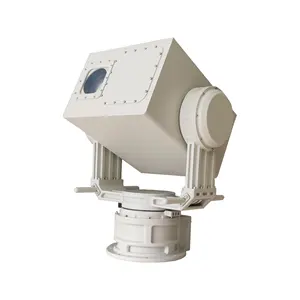This is a photo of a white, box-shaped technological device, likely a telescope. The device sits against a completely white background, devoid of any additional context. The main body of the device resembles a white shoebox, with numerous rivets around its exterior. A dark, circular lens is positioned at one end, suggesting its purpose as a viewing apparatus. The box tilts up towards the upper left corner of the image, supported by two straight arms on either side. These arms connect to a circular base, allowing the device to move up and down. This base presumably also enables a 360-degree rotation for comprehensive viewing angles. The overall structure appears engineered for precise, adjustable positioning, characteristic of observational tools like telescopes.